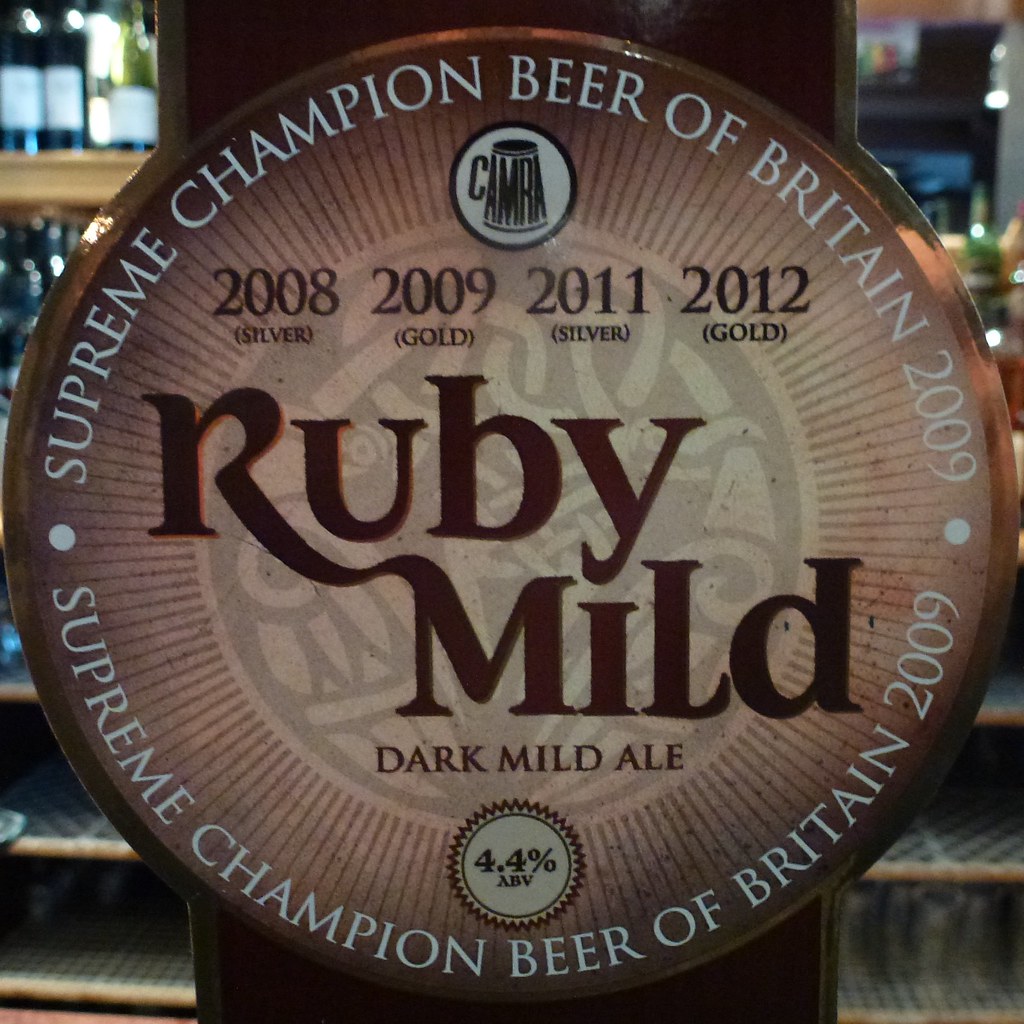This photograph features a close-up view of a circular beer sign affixed to a dark brown or red post in a bar setting. The background is blurred, showcasing shelves possibly stocked with wine bottles and glasses. The sign itself is predominantly brown, consisting of several concentric circles that transition from dark to lighter shades toward the center. Within these circles are both white radiating lines and white text that reads "Supreme Champion Beer of Britain 2009" on both the top and bottom arcs.

Dominating the center of the sign is the name "Ruby Mild," with "Dark Mild Ale" written smaller beneath it. Another circle near the bottom of the sign lists the alcohol content as "4.4% ABV." At the very top of the sign is an emblem depicting a beer mug, with "CAMRA" inscribed on it, and beneath this, the years "2008, 2009, 2011, 2012" alongside their respective awards: silver, gold, silver, gold.